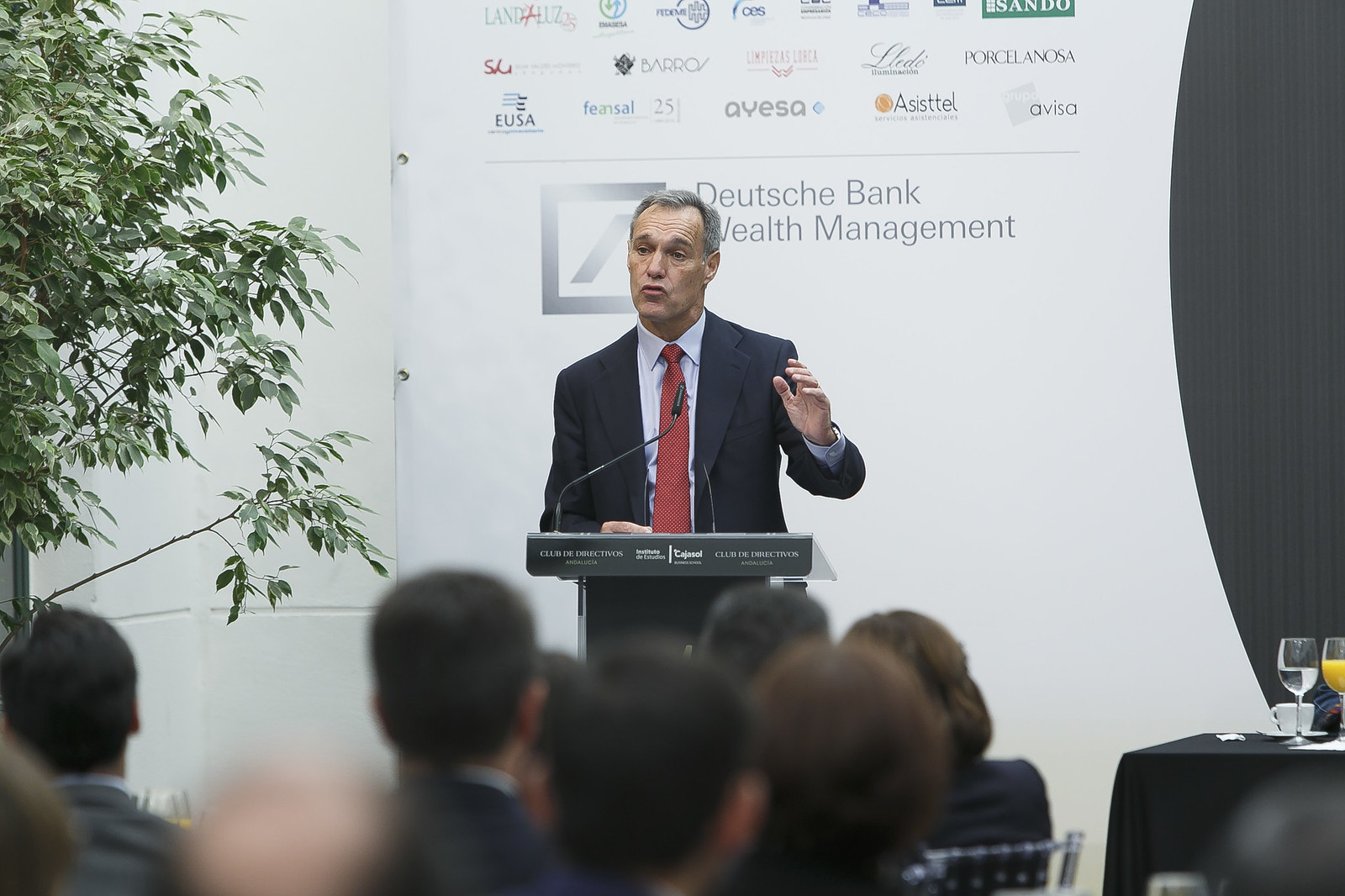In this indoor image of a speaking engagement event, an older white gentleman, dressed in a navy blue suit with a light blue shirt and a red necktie, is delivering a speech from behind a podium. He has short gray hair and is speaking into a microphone, gesturing passionately with one hand while the other rests on the podium. The backdrop displays a white banner covered with numerous company logos, the most prominent being "Deutsche Bank Wealth Management" located just behind the speaker. To his left, there is an indoor plant, appearing to be a fake tree, and to his right, a black table adorned with a glass of water and a glass of orange juice. The audience, visible from the back, is attentively seated, dressed in formal attire, and facing the speaker. The scene is framed by the professional ambiance of a well-organized, sponsor-rich corporate event.